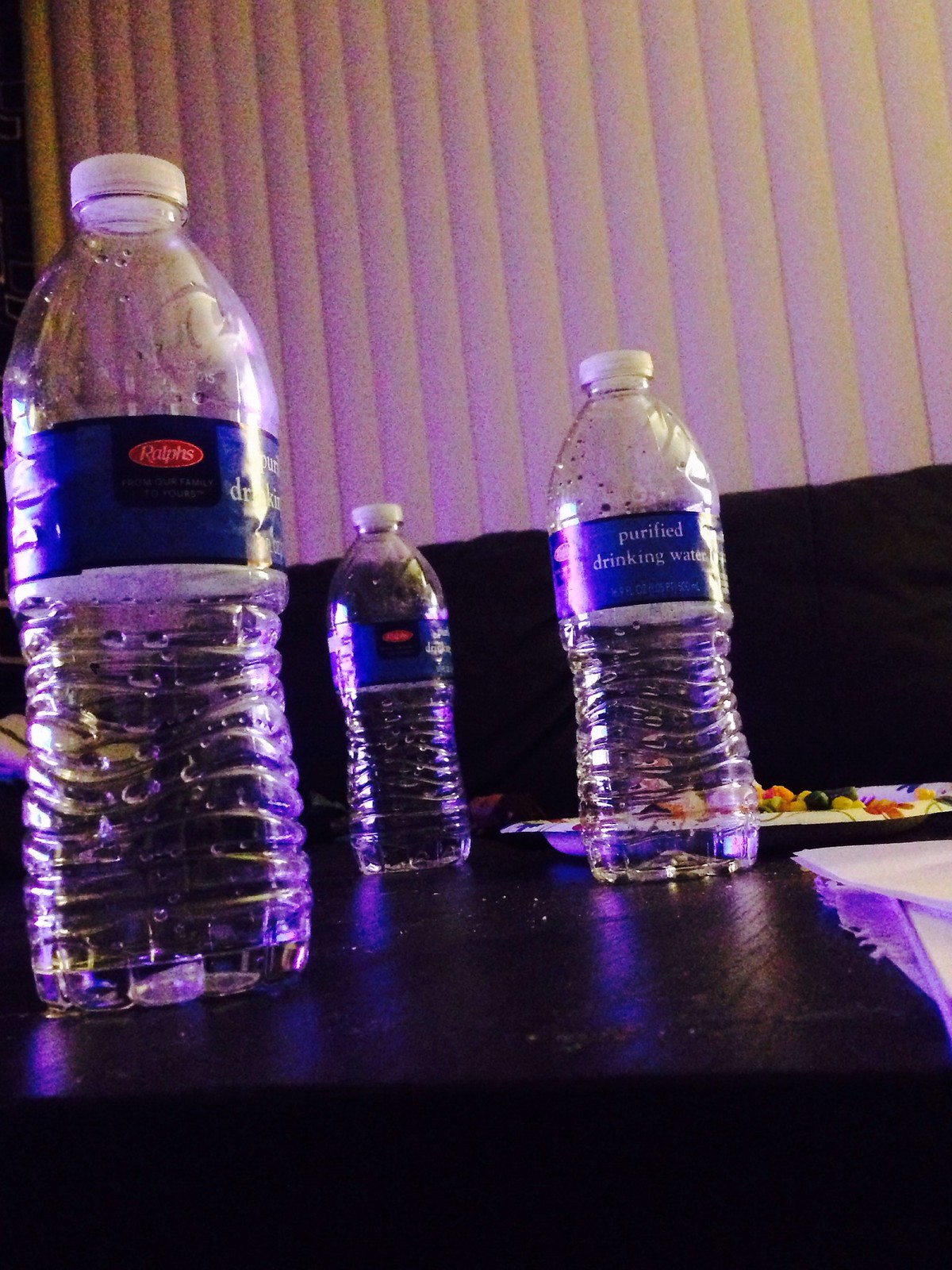The photograph depicts a dark-colored countertop or tabletop, possibly black, with light reflecting off its surface, casting subtle purple hues. Positioned prominently in the foreground are three empty plastic water bottles, each adorned with a Ralph's logo on a blue label. The bottles have white caps and the label details "purified drinking water." To the right of these bottles, there is a paper plate containing remnants of food, likely a salad with colorful ingredients such as green, orange, and black pieces. Additionally, a white napkin is partially visible in the lower right part of the photograph. The background features a very dark wall with what seems like off-white blinds or louvered shades in the upper third, allowing some sunlight to filter through.